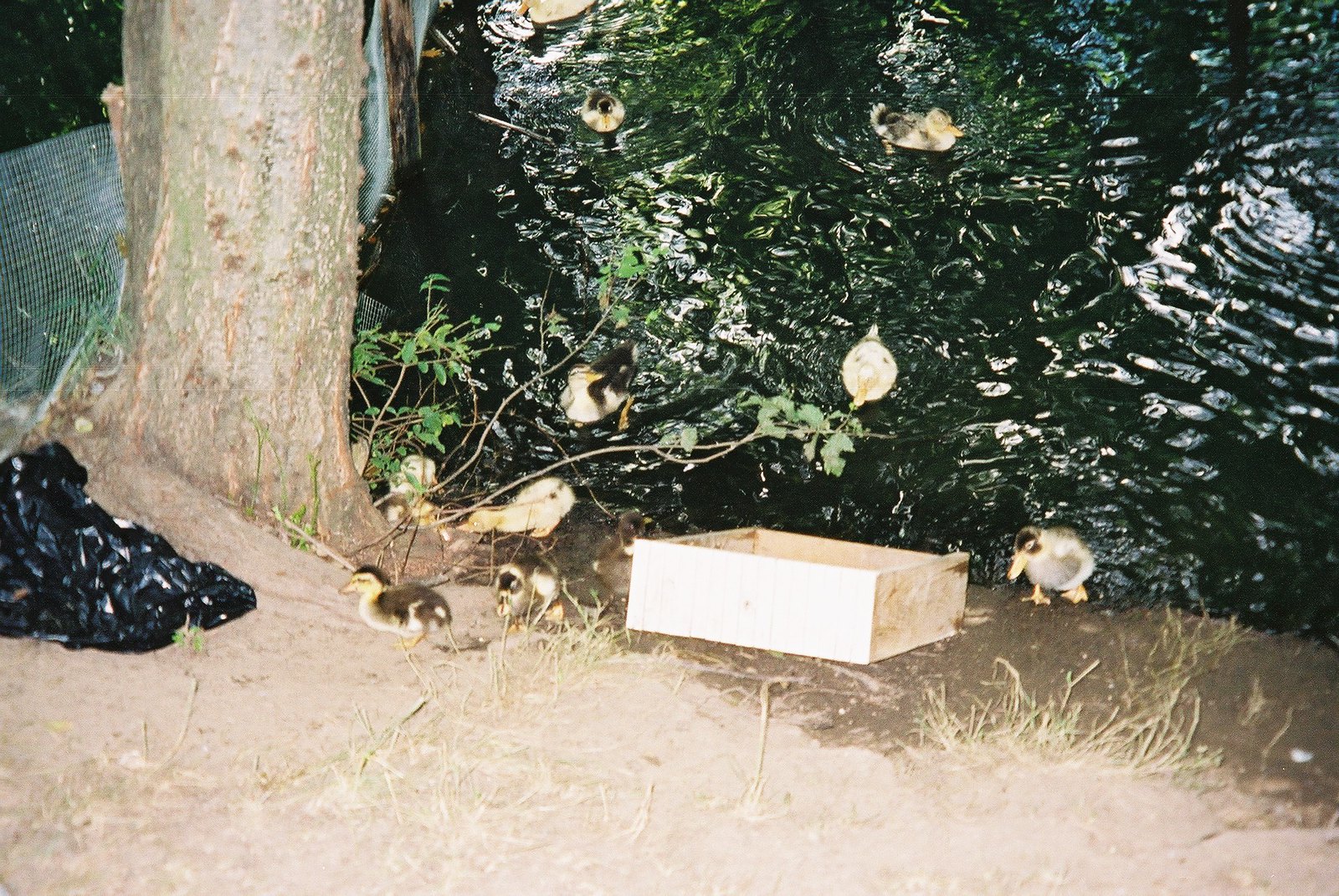The image captures a serene scene at the bank of a pond or stream, with a blend of natural and man-made elements. The focal point is a group of tiny, fluffy ducklings, predominantly yellow with touches of brown or black on their heads and backs. Several of the ducklings are swimming in the water that has notable ripples and reflections, while others are on the dirt bank, which is a hard-packed, darker brown area right at the water's edge. 

Towards the left side of the image, there is a tree with its rough, brown bark visible at the base. Near the tree trunk is a black trash bag, likely made of plastic. Adjacent to this setup and to the right of the tree is a small, shallow wooden box, slightly tilted and resting directly on the ground. The entire setting includes a sparse scattering of tufted grass and a few weeds, adding a natural touch amidst the dirt and water. 

Overall, the scene is slightly blurry, suggesting a quick snapshot, but still rich with detail, capturing the bustling, yet peaceful life along the bank of the pond or stream.